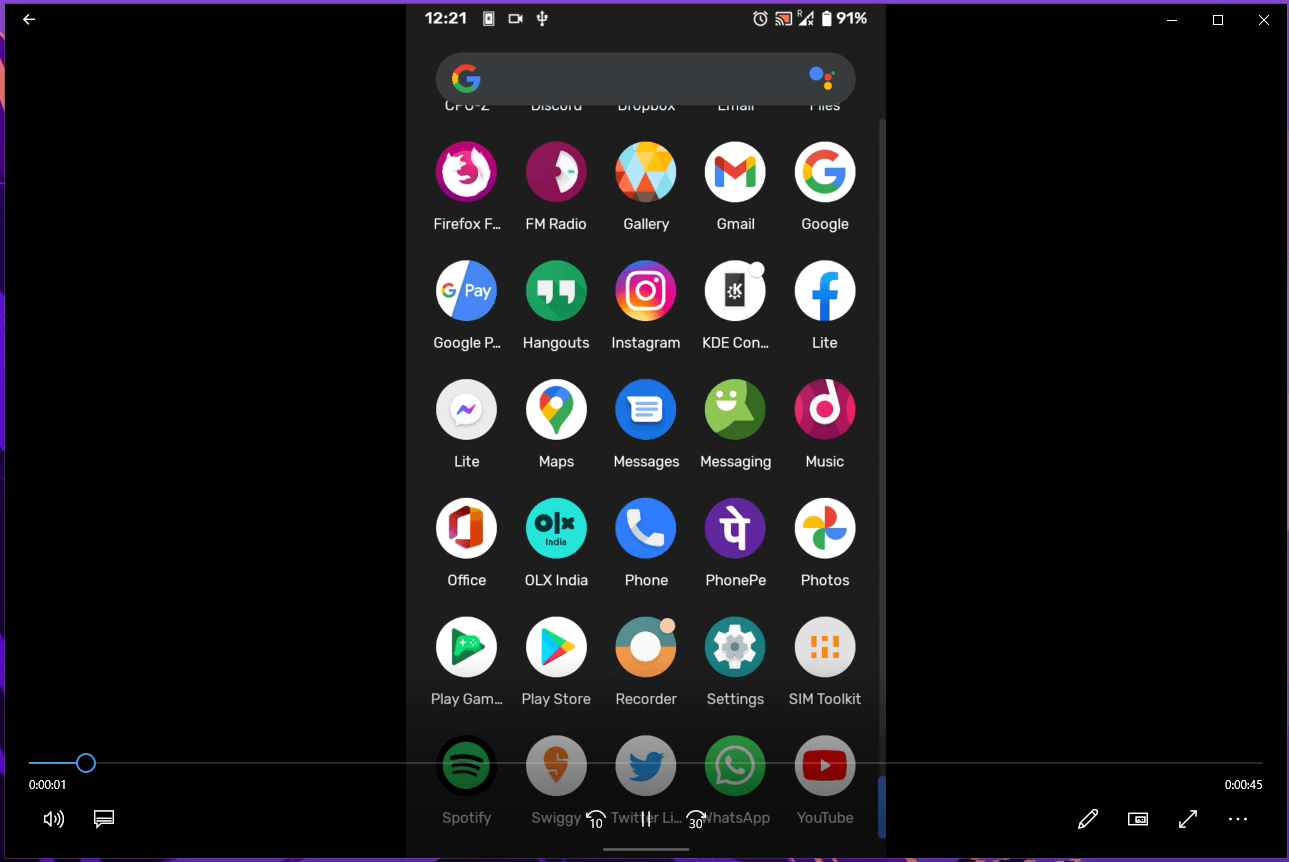A detailed caption for the provided image could be:

"A screenshot captures a phone's display showcased on a computer screen with a black background, indicating that the scene is from a video approximately 45 seconds long. The phone screen, showing a time of 12:21 and a battery level at 91%, features the Google search bar at the top, and is densely populated with icons arranged in rows of five. The visible icons include Firefox, FM Radio, Gallery, Gmail, Google, Google Pay, Hangouts, Instagram, KDE, Facebook Lite, Google Maps, Messages, Messaging, Music, Office, OLX India, Phone, PhonePe, Photos (Google Photos), Google Play Games, Play Store, Recorder, Settings, SIM Toolkit, Spotify, Swiggy, Twitter, WhatsApp, and YouTube. This screen also suggests a high level of phone activity given the numerous applications installed."